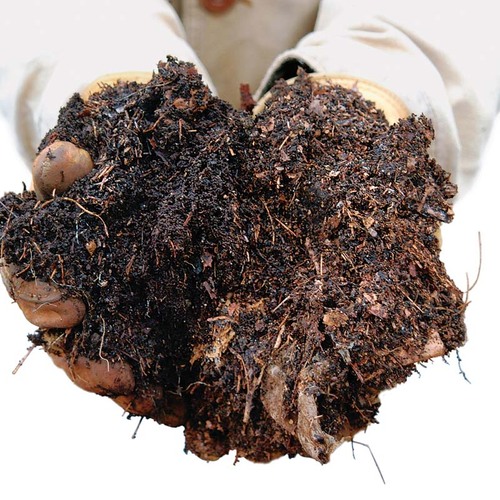In this photograph, two hands, clad in light tan gloves and extending from white long-sleeved arms, are carefully holding a large, dark, rich brown clump of compost. The compost mixture is moist and filled with various materials, including chewed-up hay, leaves, small roots, twigs, and possibly some rocks, giving it a three-dimensional appearance. The detailed, crisp image captures the person’s chest visible between the outstretched arms, but doesn't provide enough detail to determine their gender. The overall scene emphasizes the rich, earthy texture and composition of the compost, highlighting its potential as a nutrient-rich material for gardening.